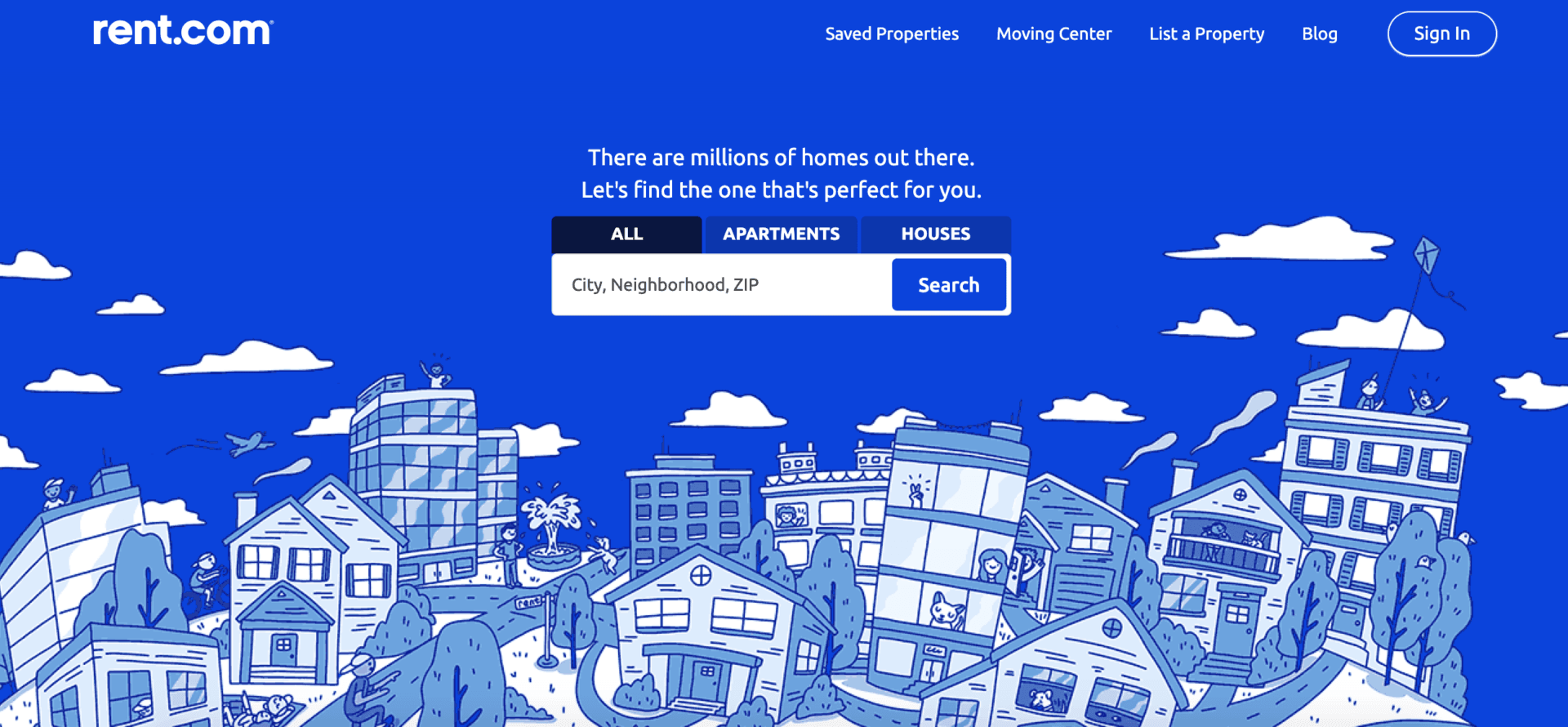The image features a predominantly blue background with the "rent.com" logo in the top left corner. In the center, an oval-shaped sign-in button stands out. Above this, a message reads: "There are millions of homes out there, let's find the one that's perfect for you." Below the message, there are options labeled "All," "Apartments," and "Houses," with input fields for city, neighborhood, or zip code. A blue rectangular search button is prominently placed.

The lower half of the image showcases a whimsical, cartoony cityscape with various building types including houses, towers, and skyscrapers. Details include clouds on both sides, diverse windows, and playful elements such as a peace sign in one window, a woman in another, a dog in yet another, and a kite being flown. There's a character cheering "yay" and roads and trees are visible on the right, adding to the lively atmosphere.